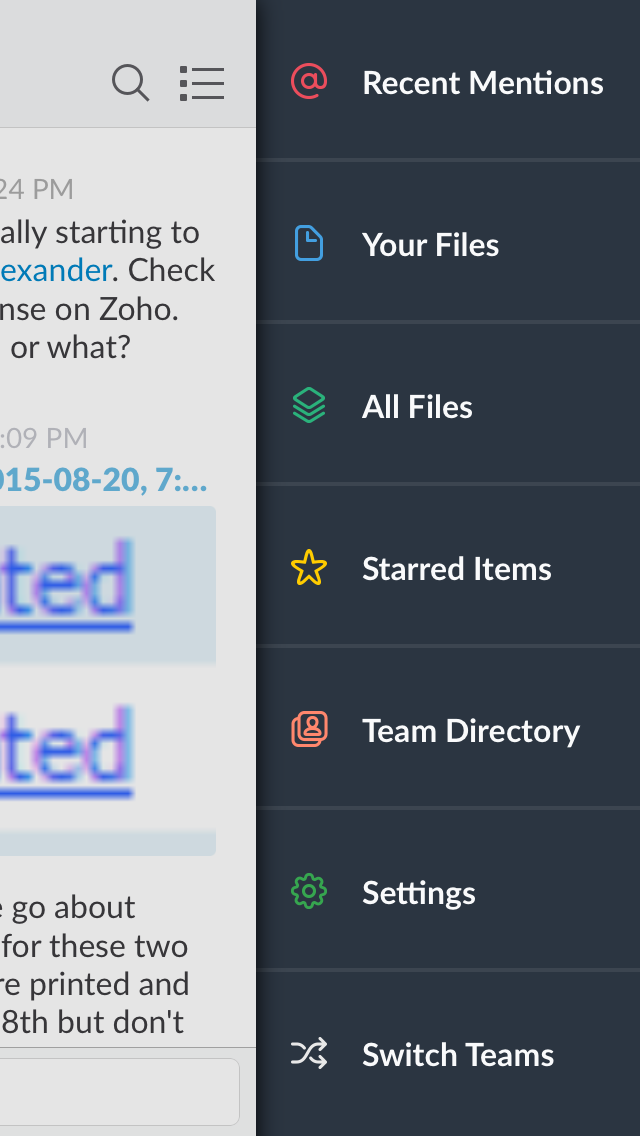This is a screenshot likely taken from a smartphone, displaying a partially visible vertical rectangular interface. On the left side, we observe a truncated list of messages where we can see only portions of the texts and times. For instance, one message shows "24" implying an hour in the afternoon (e.g., 2:24 p.m.), another shows "09" minutes past an hour (e.g., 9 minutes past). We also see text snippets like "go about," "for these two," and "printed eighth but don't," which are cut off at the edge of the frame.

To the right is a black column, a navigation bar with various headings accompanied by colorful icons. The headings and their respective symbols are:
- Recent Mentions (red at symbol)
- Your Files (blue icon of a page)
- All Files (green stack of papers icon)
- Starred Items (yellow star)
- Team Directory (icon resembling a photo frame in red)
- Settings (green gear icon)
- Switch Teams (crossing arrows icon, black with white text)

Overall, the screenshot captures a communication or file management app interface, presumably on a phone, but potentially from a tablet or computer, emphasizing the ability to navigate through recent mentions, files, and other settings with visually distinct icons.